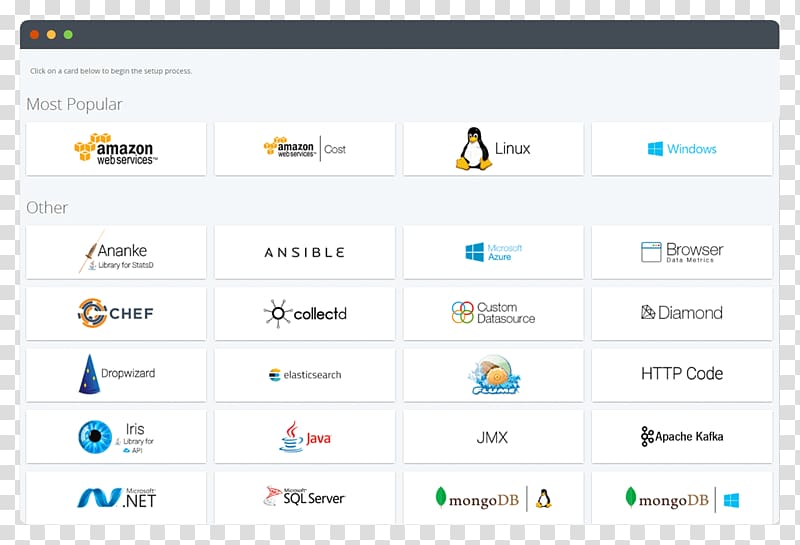The image features a sophisticated user interface design. Surrounding the image's top and sides is a checkerboard pattern in gray and white. The checkerboard covers the top border completely, and partially extends down both sides, gradually vanishing. Just inside this checkered border at the top edge is a solid black strip.

In the top left corner of the image, three colored circles are arranged horizontally: first a red circle, followed by a yellow one, and finally a green circle. Below this trio of circles, the background transitions to a light blue color. On the top left, small text reads, "Click on a card below to begin the setup process." Beneath this, larger text on the left side says, "Most Popular."

Four white rectangles span horizontally across the image, forming the first row of options. The first rectangle prominently features the Amazon Web Services (AWS) logo on the left side, followed by the text "Amazon Web Services." A vertical black line separates this text from the word "Cost." Next to the AWS card, there are icons with a penguin (representing Linux) and the blue Windows icon, denoting Windows services.

Below the "Most Popular" section is a labeled area titled "Other," on the left side. This section includes similar white rectangles organized in a horizontal layout. The design pattern continues with five rows in total from top to bottom. Each rectangle contains an identifiable company logo on the left, followed by the company name.

Overall, the well-ordered layout provides a clear and efficient interface for users to select and set up various services from a variety of companies, each represented by their respective icons and names.